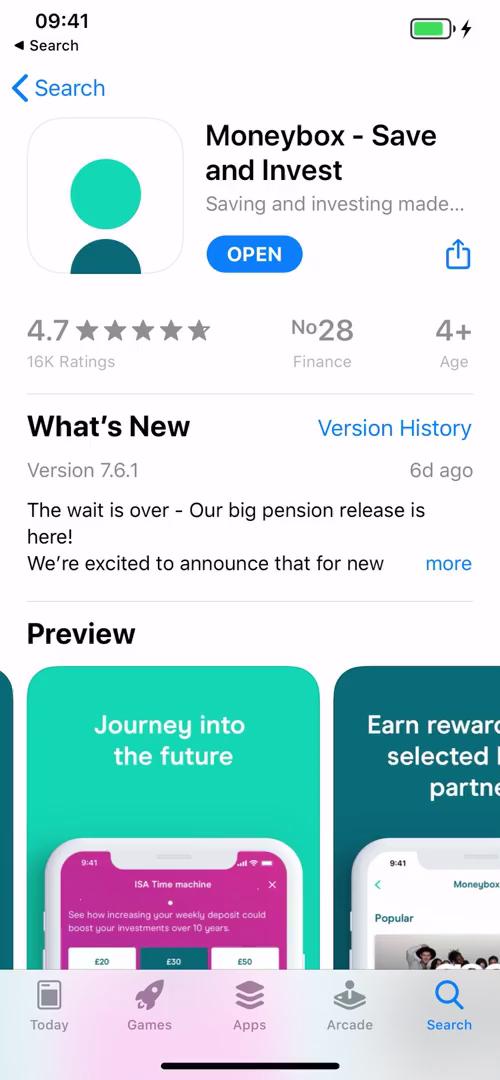Here is a more polished and detailed caption for the screenshot you described:

---

This screenshot captures the iPhone App Store page for the "Moneybox Save and Invest" app. In the top-left corner, a light blue search button and a left-pointing arrow are visible. Directly below, a large square icon representing the Moneybox app is prominently displayed. To its right, the app's full name, "Moneybox Save and Invest," is written in bold. Beneath the name, the tagline "Saving and Investing Made..." is shown in light gray text. An "OPEN" button is present below the tagline, indicating that the app is already installed on the device.

Centrally positioned on the screenshot, the header "What's New" is flanked by "Version History" on the left and "Version Histories" highlighted in blue on the right. Further down, various thumbnail images provide a preview of the app's interface, each featuring distinct colored backgrounds to visually separate them.

At the very bottom of the screen, navigation categories for the App Store are displayed: "Today," "Games," "Apps," "Arcade," and "Search." The "Search" category is highlighted in light blue, signifying the active tab.

---